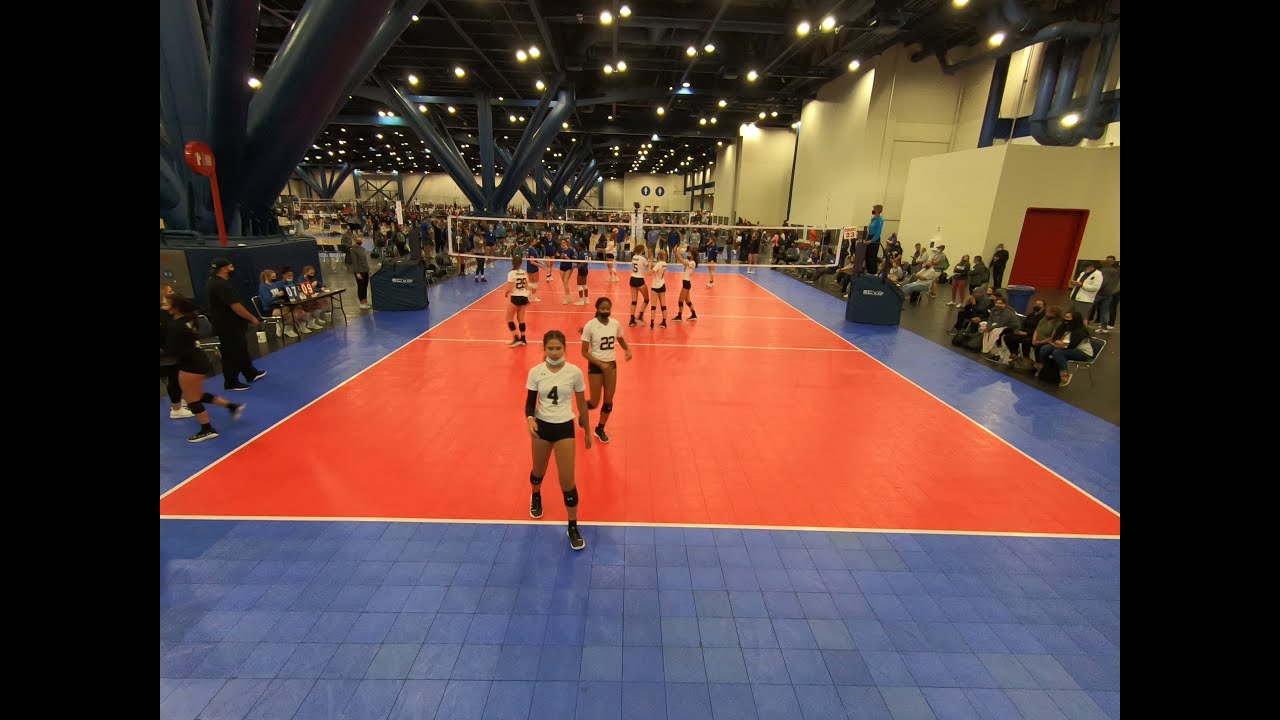The image depicts a bustling indoor gymnasium where a girls' volleyball game is taking place. The central volleyball court features a striking orange floor marked with white lines, while the surrounding area is covered with blue tiles. The young players, appearing to be around 14 or 15 years old, are split into two teams: one wearing white jerseys with black shorts, numbered prominently in black, and the other in dark jerseys with red pinstripes. The court is bisected by a net lined with white fabric, supported by dark gray poles.

Several girls from the white-jerseyed team are seen walking around the court, some grouped together facing the net, while others are moving away. A referee in a blue shirt and black pants stands by the right pole of the net, overseeing the game. Another referee, positioned on the sideline, monitors for out-of-bounds plays. Surrounding the court are numerous spectators, some seated on bleachers, others at tables, and many standing, all intently watching the match. In the expansive, yellow-walled gymnasium, additional volleyball courts and nets are visible in the background. The tall ceiling, dark blue in color with visible blue pipes and large support beams, is well-lit, highlighting the energetic atmosphere of the event.